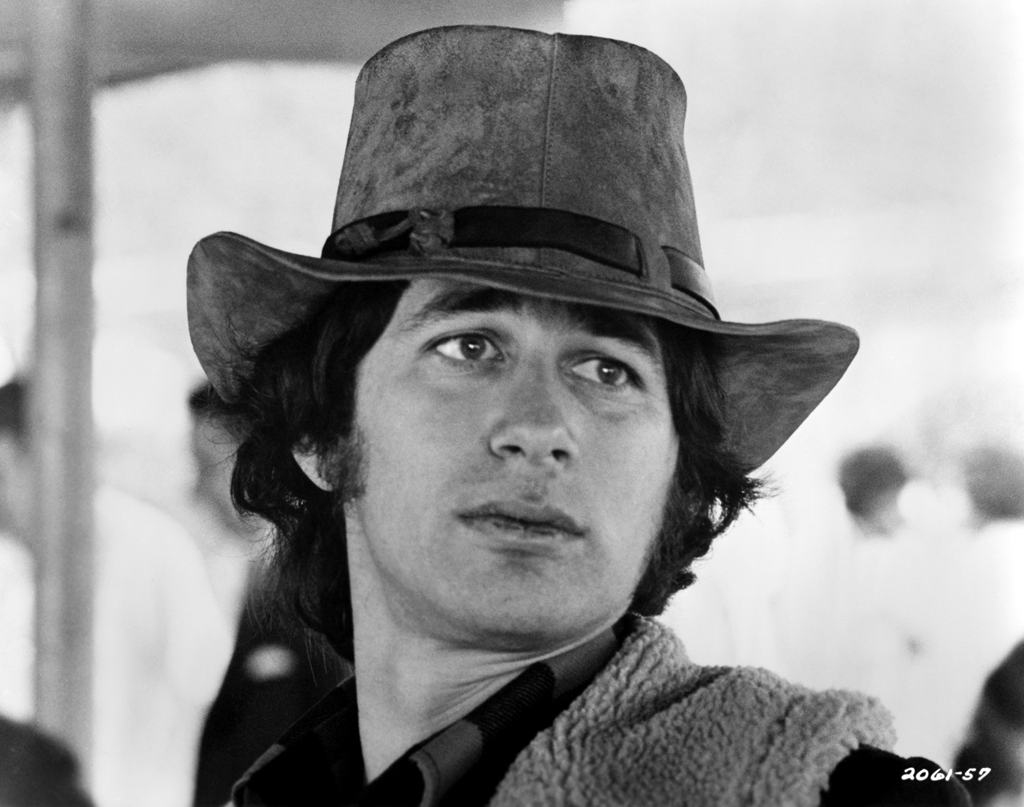The black-and-white image captures a close-up of a man, possibly an actor, seemingly during a film or TV show shoot. He is wearing a tall, felt cowboy hat with a black strap or belt across the top, and his bushy, dark eyebrows and expressive, dark eyes are prominent features. His dark, slightly shaggy hair spills out from under the hat. His expression is neutral, with his head facing slightly to the left and eyes gazing to the right. He is dressed in a collared black shirt and a fluffy cotton vest draped over his shoulders. The background is a blur of whites, grays, and indistinct figures, suggesting an indoor setting with multiple people. At the bottom right corner, the text "2061-57" is visible in white.